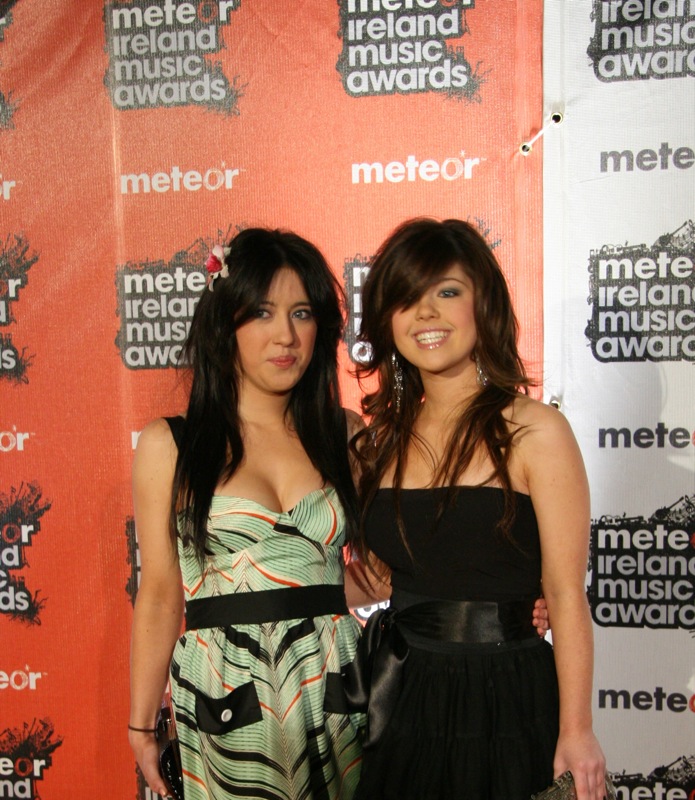In the image, two young women are posing on the red carpet at the Meteor Ireland Music Awards. The event's backdrop features alternating orange and white banners with the text "Meteor Ireland Music Awards" repeatedly displayed. 

The woman on the left has long black hair adorned with a white and red flower. She is wearing a light green dress with black and orange stripes and a black belt. Her right arm hangs naturally by her side, while her left arm is wrapped around the other woman. She holds a purse in her right hand.

The woman on the right has long brownish-red hair that drapes over her left eye and down her shoulders. She is dressed in a strapless black dress cinched with a black sash at her waist, and she sports shiny, dangly earrings. She is smiling brightly with her teeth visible, her left arm resting by her side, and her right arm around the woman in the green dress. Both women are looking at the camera, capturing the essence of the red carpet moment.